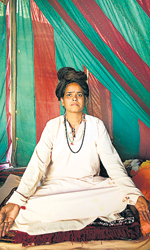In the photograph, there is a person sitting cross-legged on a layered arrangement of blankets and rugs. Directly beneath them, there is a solid red rug, followed by a brown cushion, resting on a bare floor. The individual is dressed in a long, white one-piece robe with long sleeves and an unbuttoned button-up collar. Around their neck is a black necklace, and their hair is neatly pulled up into a bun atop their head. They are holding their arms outstretched with elbows straight, palms facing forward towards the camera, giving an impression of meditation or prayer.

Behind them, the backdrop is a tent wall featuring alternating vertical stripes of green and red, with a portion of the same striped fabric draped diagonally across the upper right corner of the image. To the person's right, additional cushions and blankets are visible, including a black cushion adorned with blue and yellow floral patterns and a bundled-up orange blanket. Although the individual's facial expression is neutral or slightly frowning, giving a sense of seriousness, the detailed surroundings create a rich and layered scene.